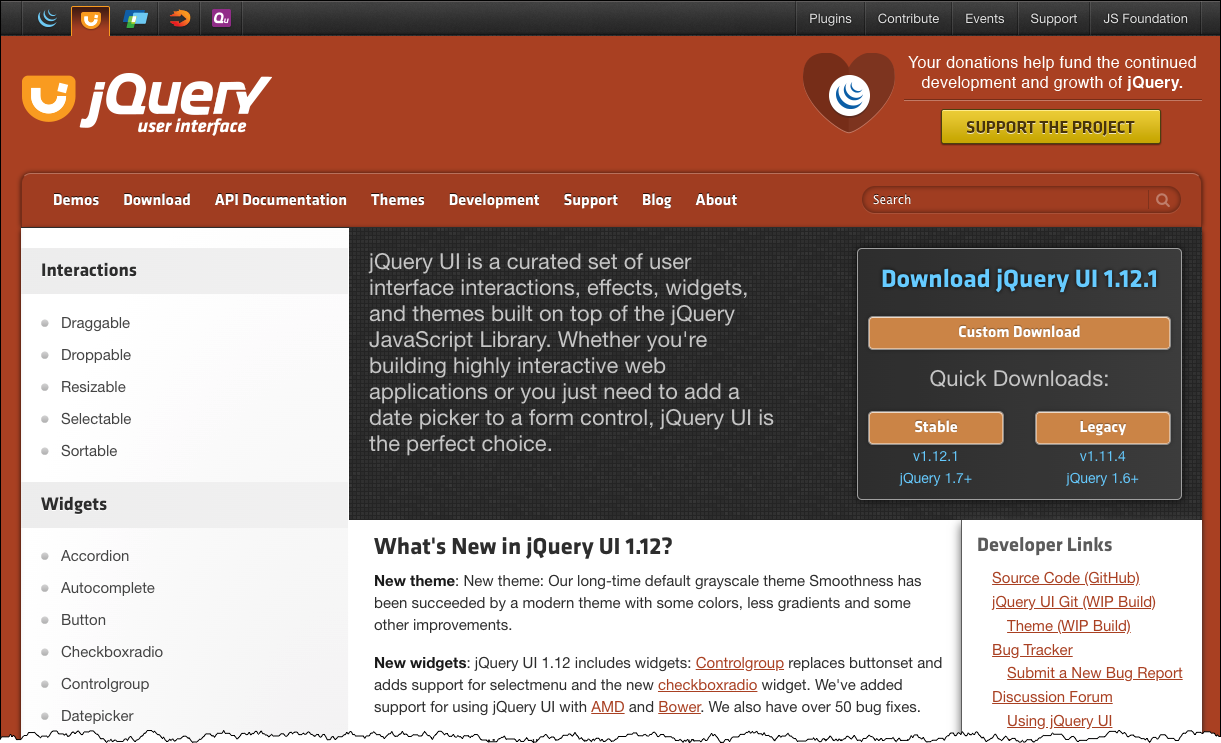Screenshot featuring a red background with various UI elements and informative text about jQuery. At the top, bold letters spell out "jQuery" with a capital "Q." A heart icon and a circle with three blue lines are displayed nearby. The text highlights the importance of donations with a message in white: "Your donations help fund the continued development and growth of jQuery." 

A prominent yellow rectangle encourages users to "Support the Project." Navigation options are available for "Demos," "Download," "API," "Documentation," "Themes," "Development," "Support," and "Blog," along with an "About" section and a search bar. Interface functionalities are listed, including "Interactions" (draggable, droppable, resizable, selectable, sortable) and "Widgets" (accordion, autocomplete, button, checkbox, radio, control group, datepicker).

For downloads, the text "Download jQuery UI 1.12.1" is highlighted in blue, along with an orange rectangle that offers a "Custom Download" button in white.